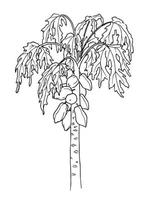This is a detailed, black and white, hand-drawn sketch of a coconut palm tree, approximately one inch by one inch in size. The drawing features a thin trunk with visible marks or specks near the base. At the top of the trunk, several large, lobed palm fronds extend outward. There are three fronds on the left side and around four to five on the right side, elegantly bending and draping down. In the center of the fronds, a cluster of coconuts is depicted, with one prominently round coconut and several oblong-shaped coconuts—totaling about eight or nine pieces. The detailed line work is possibly done in pencil or pen and lacks any shading or background, focusing solely on the tree itself. Intriguingly, the arrangement of coconuts and fronds hints at a subtle, artistic style possibly evoking other elements, but it's definitively a simple and expressive representation of a coconut palm tree.